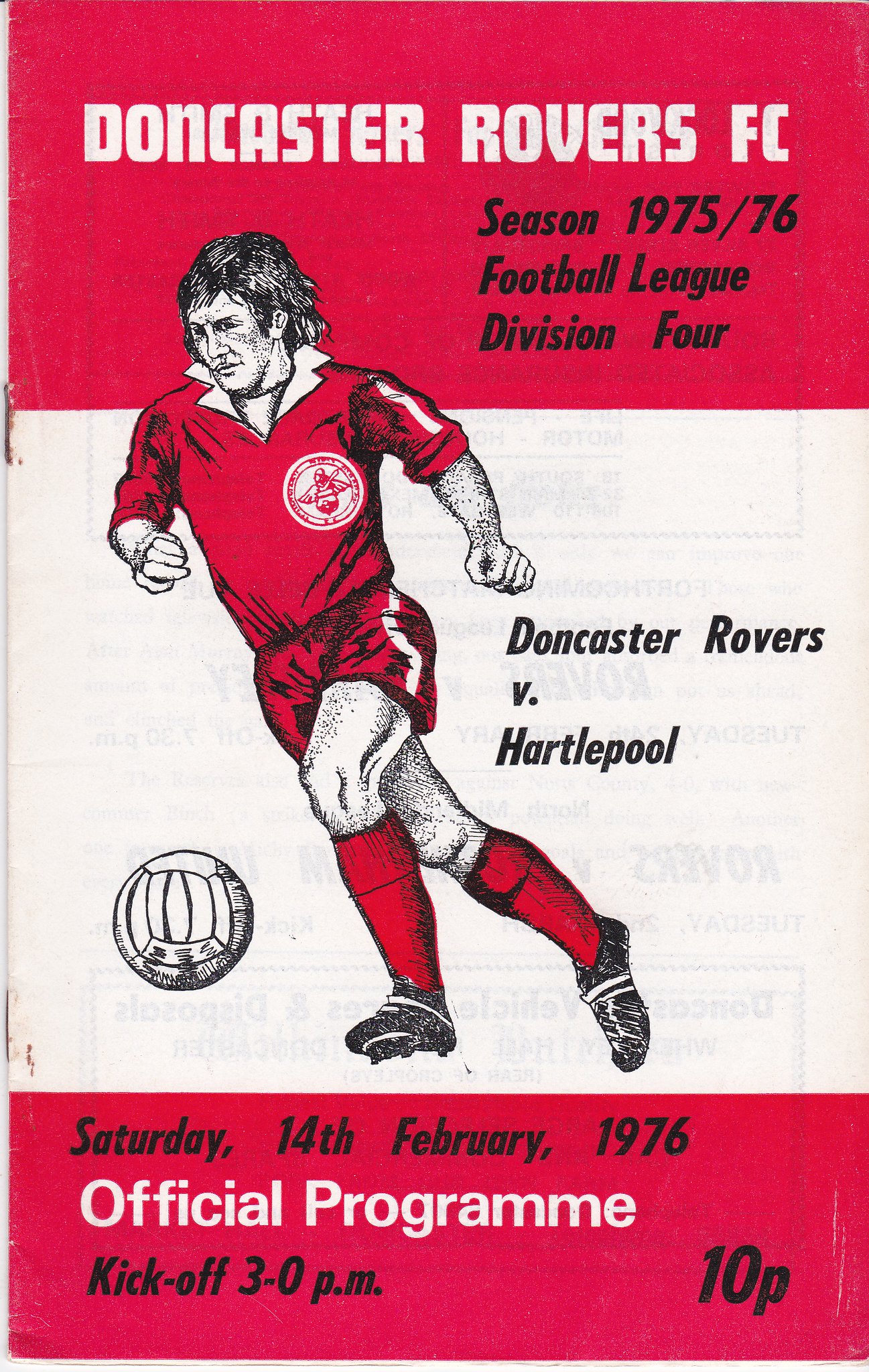The image depicts the front cover of a football program, divided into three color-blocked sections: red at the top and bottom, and white in the middle. The top red section features "Doncaster Rovers FC" in bold white print, with "Season 1975-1976" in black letters to the right. Below this, the text reads "Football League" and "Division Four." 

In the white middle section, the right side announces the match-up, "Doncaster Rovers vs Hartlepool." Dominating the left side and extending from the top red area to the bottom of the white region is a sketch of a soccer player in a red shirt with white stripes on the sleeves, red shorts with white stripes, and red stockings. The player has short dark hair and is depicted in motion with a soccer ball in front of him.

The bottom red section includes more details: "Saturday, 14th February 1976" in black, "Official Program" beneath it in white, and "Kickoff 3:00 p.m." Black text in the bottom right corner marks the price as "10p." Overall, the cover integrates detailed thematic and visual elements, emphasizing the event and team spirit.